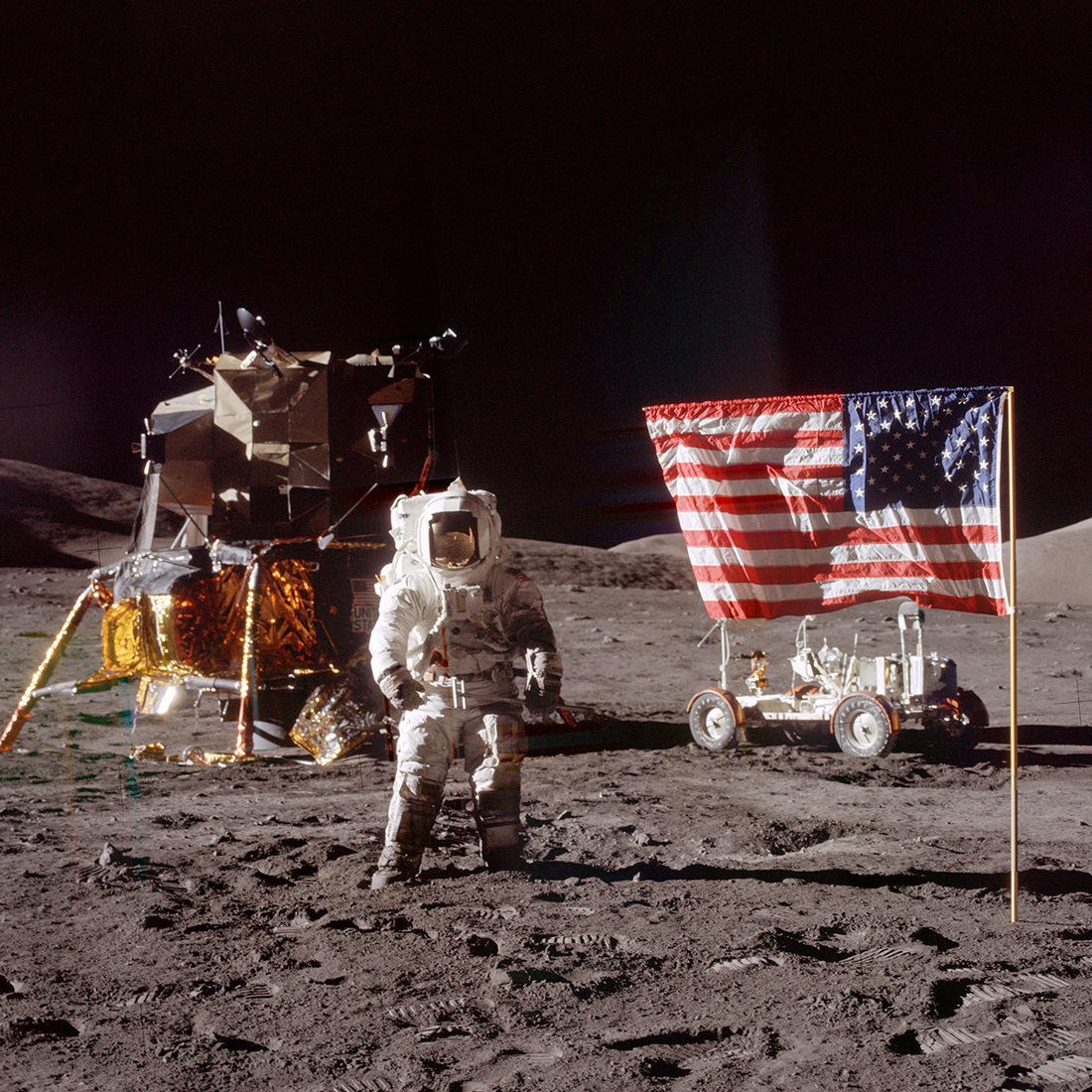This is a perfectly square, color photograph of an astronaut on the moon, capturing an iconic moment from the moon landing. The top half of the background is a pitch-black sky, while the bottom half is the moon's surface, depicted in varying shades of gray and charcoal. Footprints from the astronauts are visible across the surface. At the center of the image stands a lone astronaut in a full space suit with a reflective golden visor on the helmet. To the right, the American flag with its blue field and white stars and red and white stripes flutters, and beneath it is a white lunar rover with dark wheels. To the left, behind the astronaut, a spacecraft landing module with a base covered in shiny gold foil and supported by sturdy legs, stands proudly. The scene is devoid of any other people or text, focusing solely on the astronaut, the moonscape, and the artifacts of human exploration.